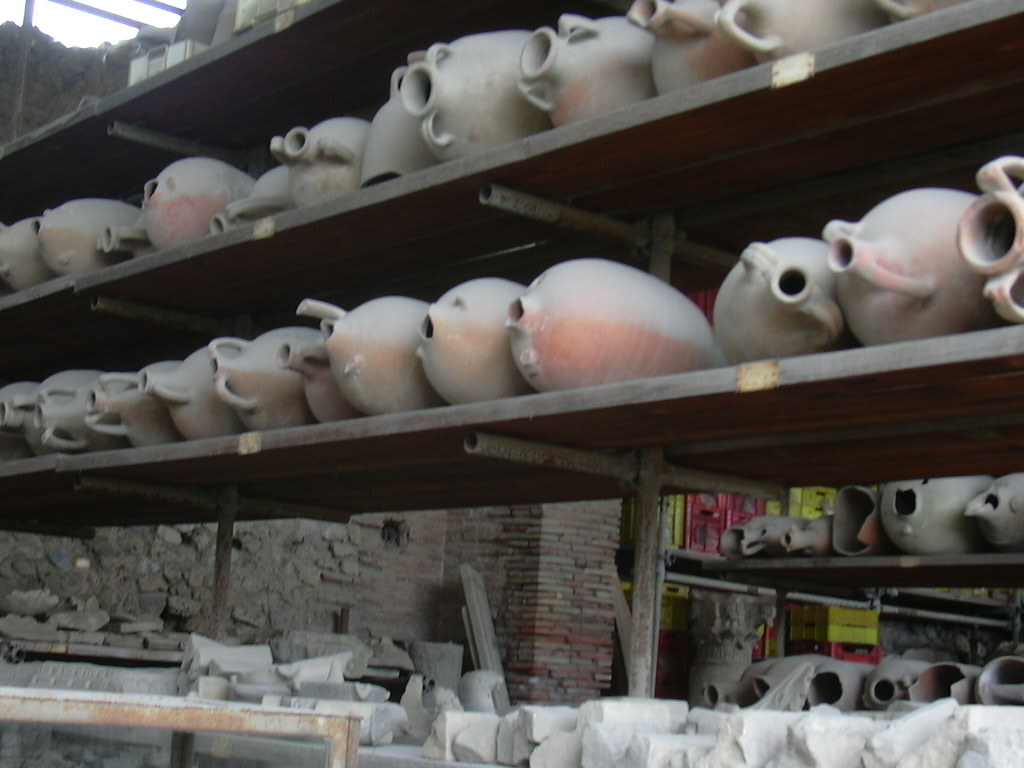This photograph captures a large, somewhat cluttered pottery workshop, characterized by industrial dark-brown shelving units that are filled with various ceramic pieces. The main focus is on three main shelves: the top shelf, partially obscured, the middle shelf, and the bottom shelf.

On the middle shelf, several unglazed terracotta and clay jugs are prominently displayed. These jugs are predominantly reddish-orange in color, though many exhibit a dusty or whitish haze that suggests they've been there for a while. Their designs are varied, with some jugs showing signs of damage, such as broken handles or irregular mouths. The vases and jugs appear round and tall, often with one or two handles near their narrow openings. Many of them are also lying on their sides, with their openings facing outward toward the viewer.

The bottom shelf is similarly packed with more pottery pieces, including additional jugs, some of which are covered in dirt. These pieces are stacked haphazardly, suggesting a busy workshop environment. Below this shelf, part of the storage might include white, brick-like shapes, possibly either stones or unfinished pottery projects.

In the background is a worn brick wall, comprising both large old bricks and smaller bricks forming a chimney. Alongside this, there are red and yellow crates, adding a pop of color to the otherwise muted scene. The overall appearance of the space hints at it being an outdoor or semi-outdoor workshop, with a portion of the sky visible in the upper left corner of the image. The setting, with its lines of shelves extending back into the room, conveys a sense of depth and a busy, industrious atmosphere.